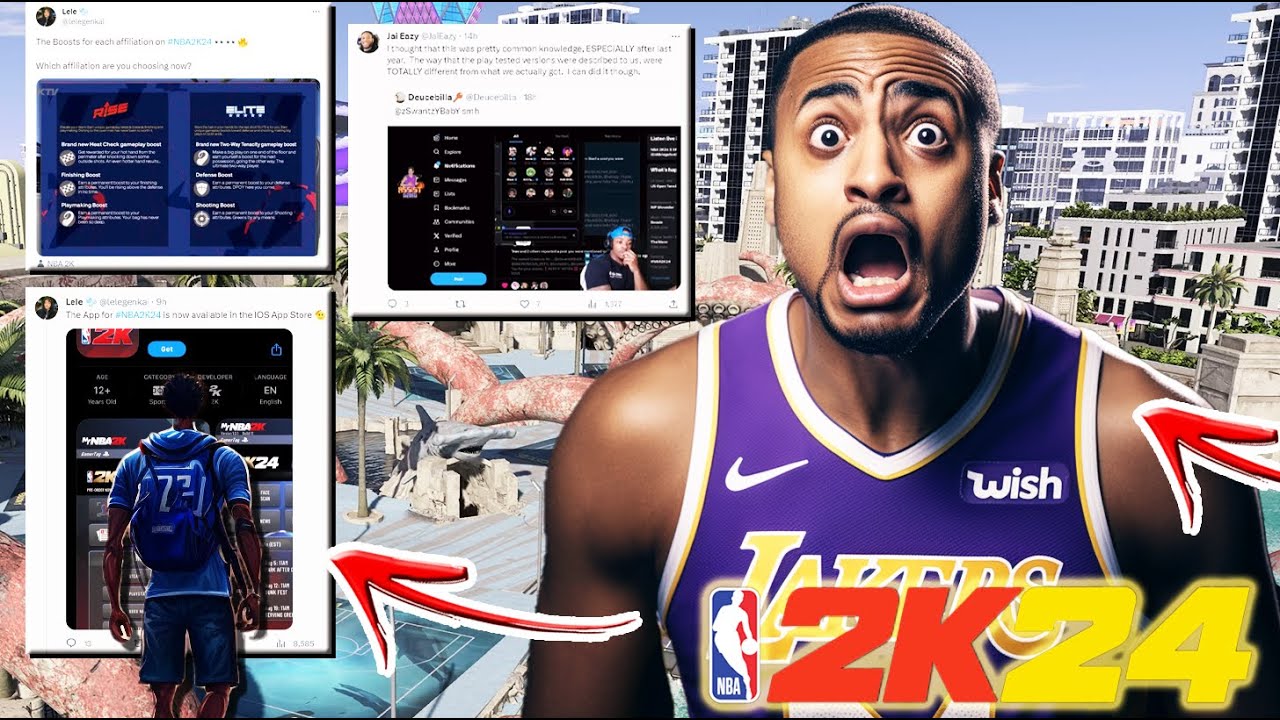A vivid scene capturing a luxurious resort complex, featuring high-rise condos with balconies and statues nestled amidst tropical palm trees. The blue sky and expansive swimming pool, complete with a faux shark and decorative rocks, provide a serene setting. On the left side of the image, screenshots from what appears to be a game tweet can be seen. One screenshot depicts a character with their back to the camera, dressed in a blue shirt, blue shorts, and a matching backpack, with a red arrow indicating their direction. Another screenshot shows a basketball player in a Lakers jersey, seemingly shouting at the camera, also marked by a red arrow. The text "2K24" is visible at the bottom of these images, suggesting they're related to the video game NBA 2K24. The image juxtaposes the calm of the resort with the dynamic energy of the game, creating an intriguing visual contrast.